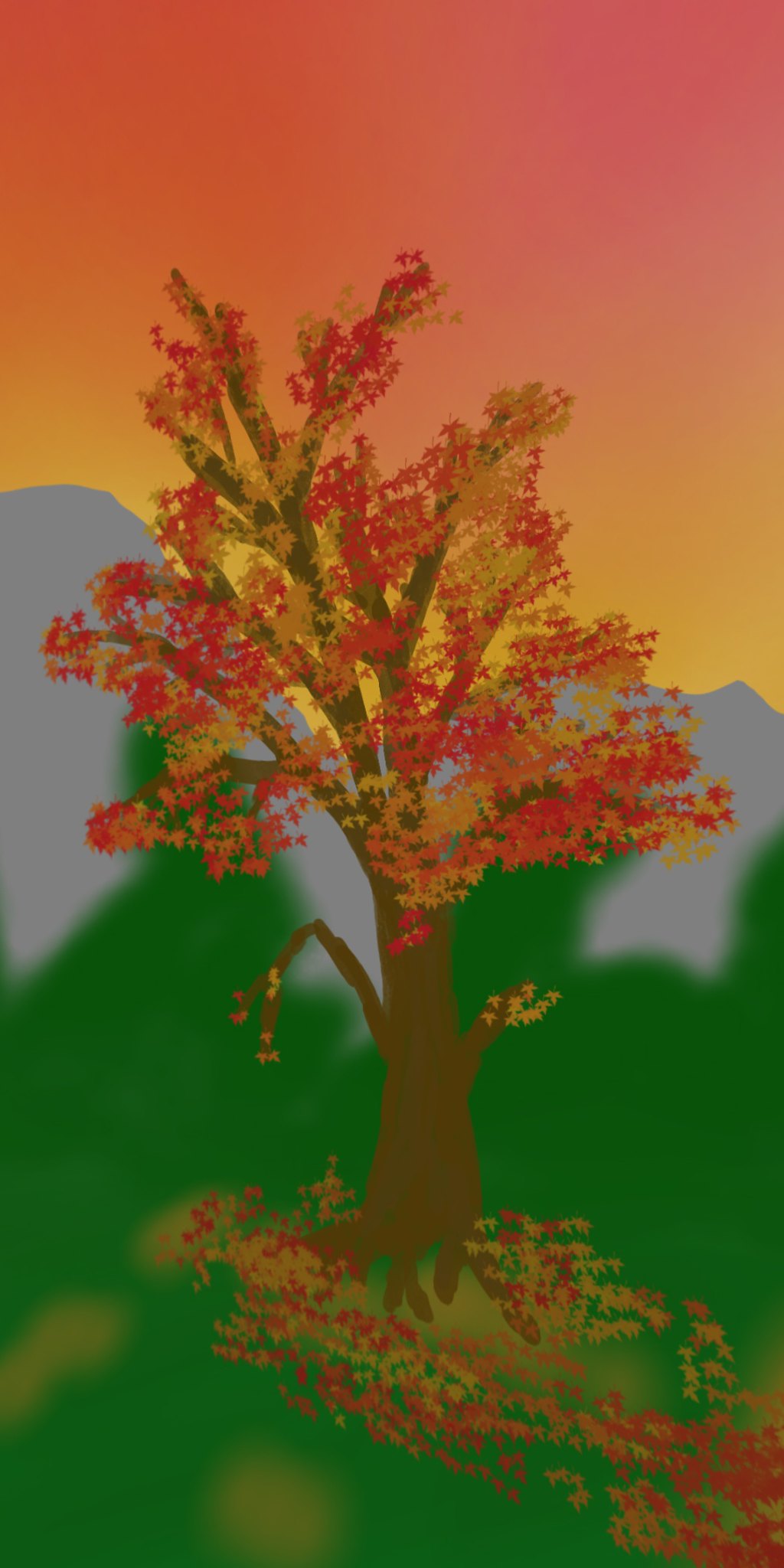This hand-drawn image presents a central tree that dominates approximately two-thirds of the frame. The tree's bark is a sturdy brown, with gnarled roots visible at the base. Its foliage is a vibrant medley of autumn hues, including yellow, light orange, dark orange, and red leaves, giving the tree a rich and dynamic crown. Extending from the left side of the trunk is a downward-facing branch adorned with a blend of yellow, orange, and red leaves. A smaller, thicker branch emerges from the right side, bearing yellow and orange leaves.

The area around the base of the tree and the ground is speckled with fallen leaves in shades of yellow, orange, and red, creating a colorful, scattered carpet. The bottom third of the image depicts a green ground with yellow splotches, particularly noticeable on the bottom left and beneath the tree. The middle third features a serene gray-blue background accented with patches of green. The top portion of the image transitions into a sunset palette, blending hues of yellow, purple, and orange, which casts a warm, tranquil glow over the entire scene.